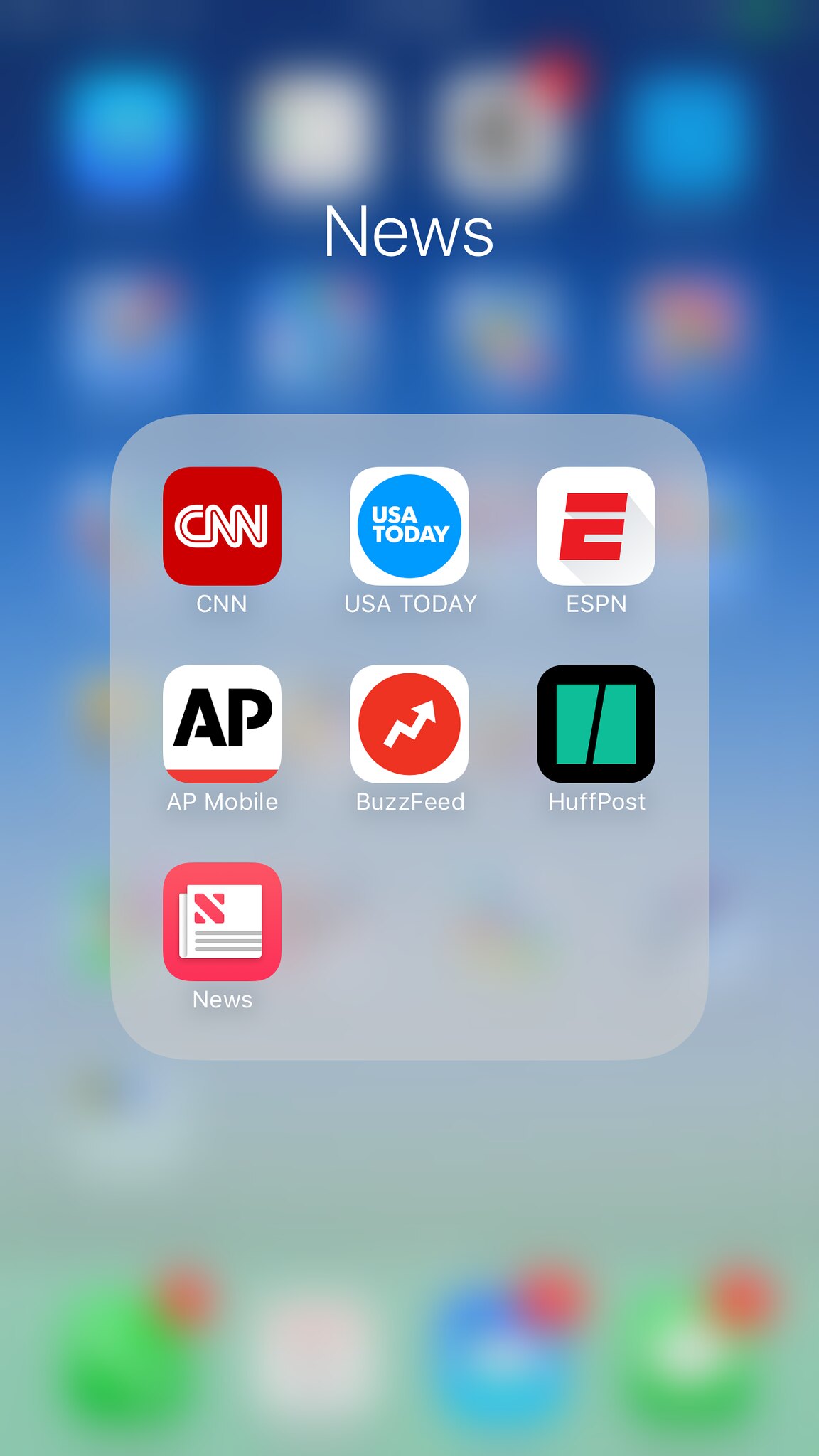This is a portrait-oriented screenshot of an iPhone home screen. The primary focus is a grey folder labeled "News" in white font. Inside the folder, there are two rows and a single app at the bottom in the third row.

- The first row contains: CNN, USA Today, ESPN, and Neatum.
- The second row includes: AP Mobile, BuzzFeed, and HuffPost.
- The third row has: Apple News.

The background of the image is fully blurred, revealing only the structure of five vertical rows of apps arranged in four columns. At the bottom of the image, the blurred home bottom bar is visible, featuring the commonly used apps including Phone (with a red notification dot), Calendar, Mail (also with a red notification dot), and Messages (with a red notification dot).

The top row of the apps on the home screen shows the third app from the left also has a notification (red dot) above it. All these details are subtly blurred, drawing attention predominantly to the "News" folder.

Overall, the screenshot represents a neatly organized iPhone home screen with a focus on news-related apps.